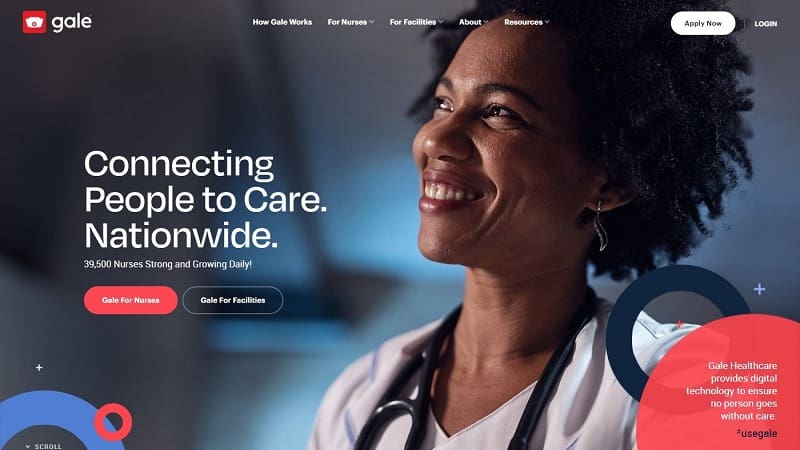This horizontal image depicts a website interface, likely accessible via computer or smart devices. The background features a photograph of an African American woman, presumably a medical professional, smiling and looking slightly upwards to the left. She is adorned in a white lab coat with a black stethoscope draped around her neck. At the top of the image, the name "Gail" is prominently displayed along with a small icon to the left of it. Central to the image are tabs labeled "How Gail Works for Nurses," "For Facilities," "About," and "Resources," suggesting a focus on healthcare services.

To the top right are buttons enabling users to "Apply Now" or "Log In." Bold white text towards the left side of the image reads, "Connecting people to care nationwide," with a subtler message underneath stating, "39,500 nurses strong and growing daily." Below this, there are options to either explore "Gail for Nurses" or "Gail for Facilities," both indicated by clickable red buttons.

In the bottom left corner, a blue semicircle slightly overlaps the edge of the frame, while the bottom right corner contains a nearly cut-off dark gray circle with a lighter center holding a plus sign. Adjacent to this is a partially visible red circle. The text within the image promotes Gail Healthcare, noting: "Gail Healthcare provides digital technology to ensure no person goes without care. Use Gail."